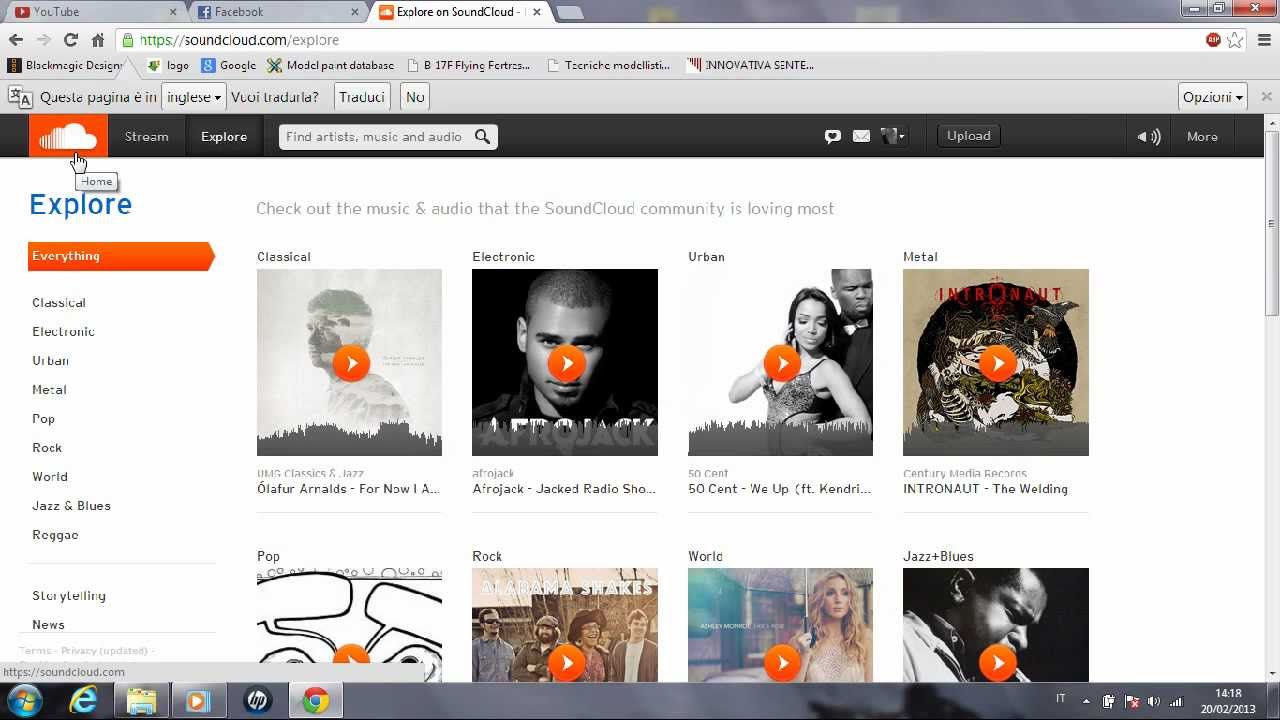A screenshot displays a web browser with three open tabs at the top: YouTube, Facebook, and SoundCloud. The SoundCloud tab is active, characterized by its signature orange background and a small cloud logo. The sidebar on the left offers categories for exploration, including Classical, Electronic, Urban, Metal, Pop, Rock, World, Jazz, and Reggae. Beneath these options, there are additional choices labeled "Explore," "Google," and "HP Folders." The bottom of the sidebar presents eight selectable squares, each corresponding to different music genres like Classical, Electronic, Urban, and Metal. The interface is neatly organized, and a small play button is visible, allowing the user to listen to tracks. There are no specific groups or artists highlighted in this view, but the functionality for navigation and music discovery is clearly emphasized.